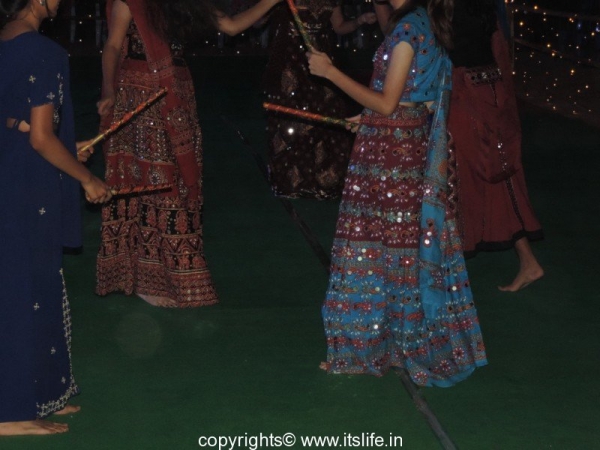The photograph captures a vibrant dance performance, possibly at an indoor event, featuring five barefoot women standing on a green astro turf. The background is a solid black wall speckled with dots that resemble a night sky filled with stars. All five women are dressed in colorful saris, each adorned differently. Notably, the woman on the far left, dressed in a blue sari with white stars, is facing the top right corner and holds two sticks wrapped in red and green ribbons, one in each hand. Two other women in the image are also holding similar ribbon-wrapped sticks. Three of the women wear red and golden saris, while the central figure dons a sari with intricate rows of blue and red decorated with gems and flowers. The performers are arranged centrally in the frame, lending focus to their rhythmic movements and traditional attire. At the very bottom of the image, white text reads "copyright www.itslife.in," marking the photo's origin.